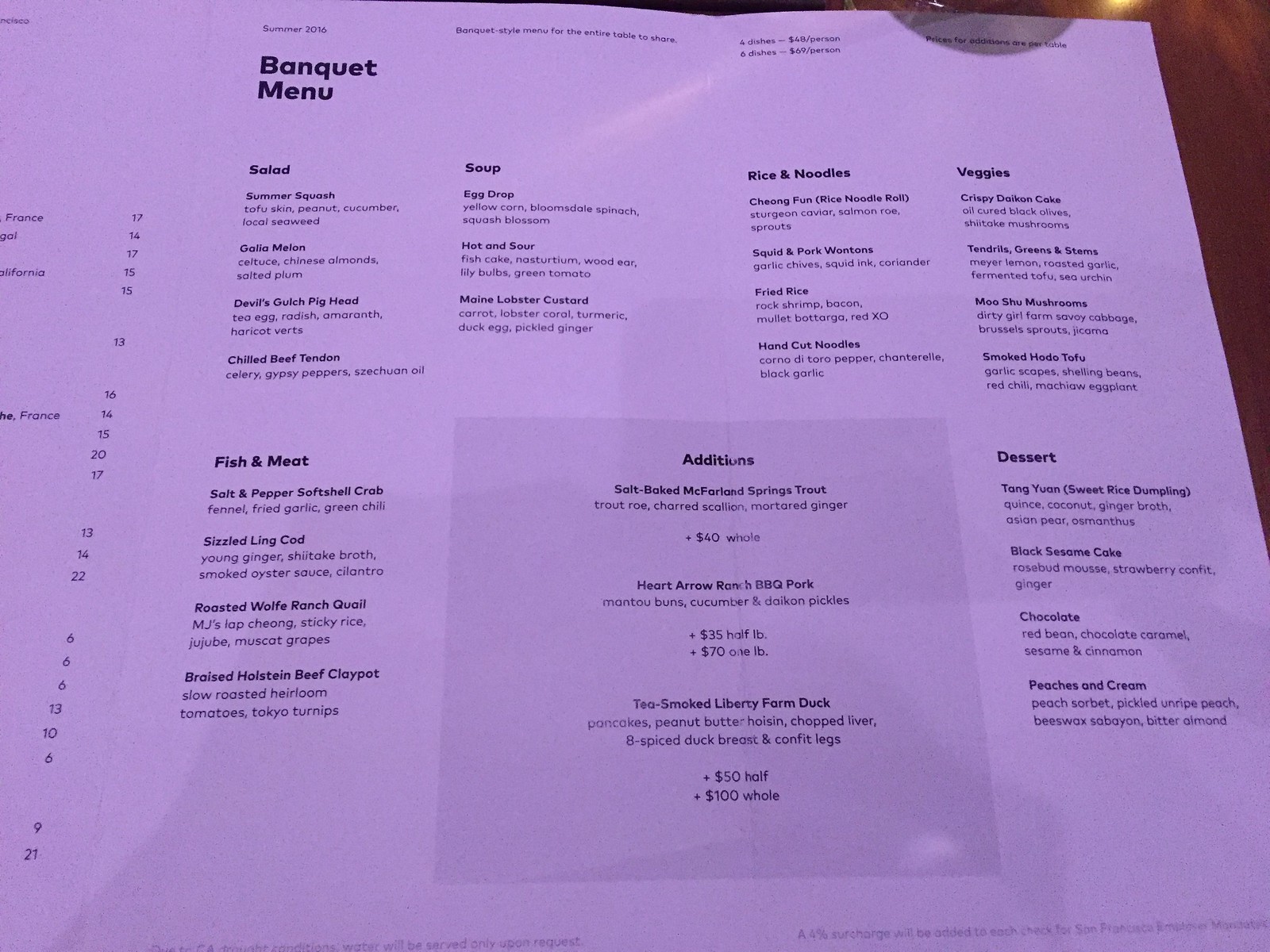The image, captured in landscape format, presents a banquet menu titled "From Summer of 2016" against a light purple background. The menu is meticulously organized into four columns, each specifying different categories of cuisine. 

In the first column titled "Salads and Fish & Meat," a variety of unique dishes are listed: summer squash, Galia melon, devil's goat, pig's head, and chilled beef tenderloin for salads, followed by salt and pepper soft-shelled crab, sizzled green cod, roasted wolf ranch quail, and braised Holstein beef claypot under fish and meat.

The second column is dedicated to "Soup," featuring egg drop soup, hot and sour soup, and Maine lobster custard.

The third column encompasses "Rice and Noodles," offering chung fun (rice noodle rolls), squid and pork wontons, fried rice, and hand-cut noodles.

The fourth column, "Veggies and Dessert," includes dishes like crispy Dahlian cake, tendrils, greens and stems, mushu mushrooms, and smoked fondo tofu. For dessert, the menu lists hang yuan, black sesame cake, and chocolate and peaches.

Centrally positioned between the middle two columns is a section entitled "Additions," slightly grayed out to distinguish it from the rest of the menu.